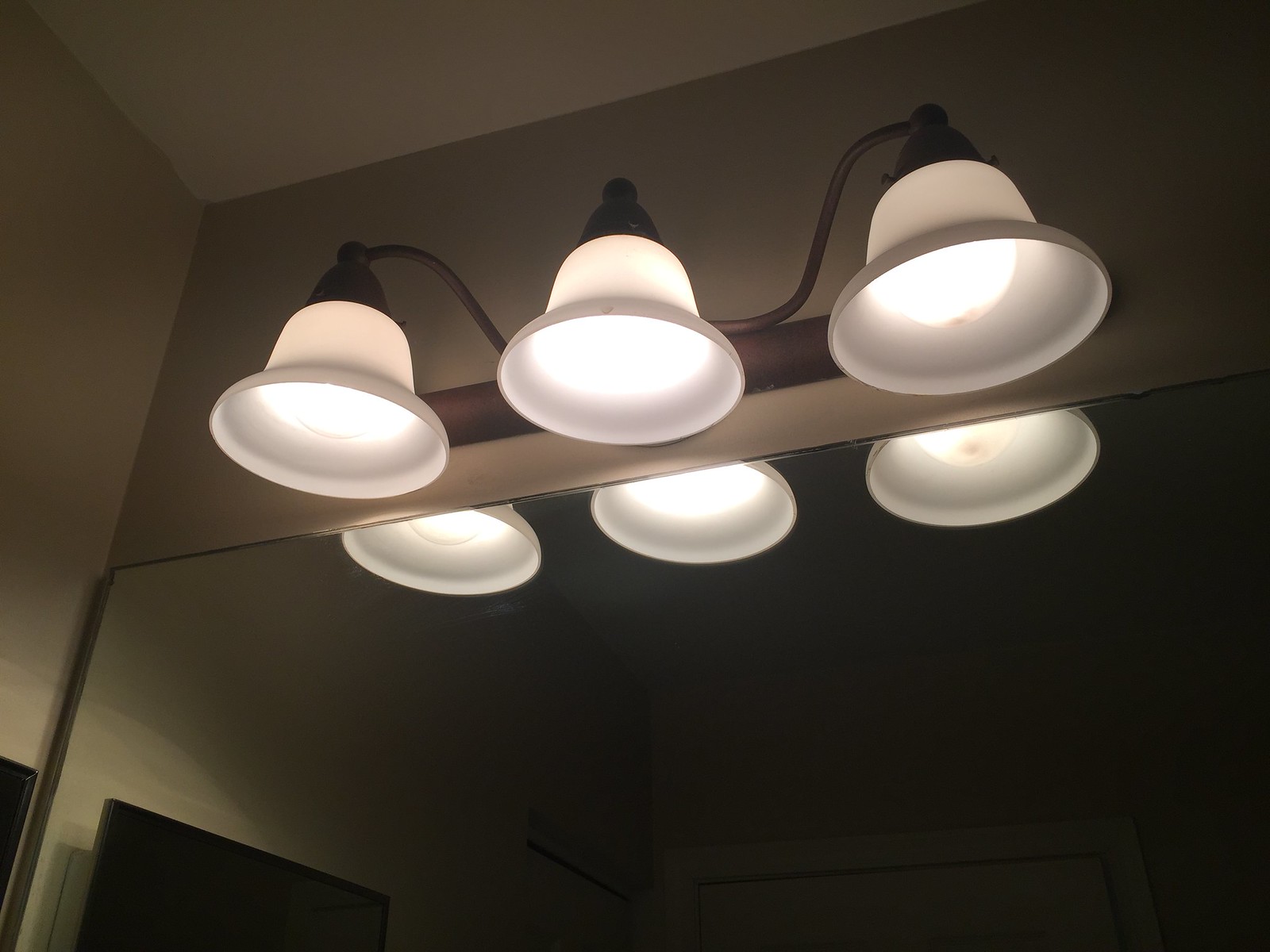This dimly lit, color photo captures the upper corner of a room with dark gray painted walls and a white ceiling. The focal point of the image is a white light fixture attached to the wall, featuring a weathered metallic brown base with three bright, bell-shaped lights. Each light has a milky frosted white shade and a rounded brown finial. The lower part of the image reveals a wide glass mirror, which reflects the rest of the room including the three illuminated lights and their bulbs. The mirror also shows two white-bordered doorways and a framed picture on the left side. In the lower left corner of the photo, there is a small part of a black square shape, possibly a TV screen. The overall composition gives an impression of looking upwards at the light fixtures, with six lights visible in total, three on each side of the mirror.